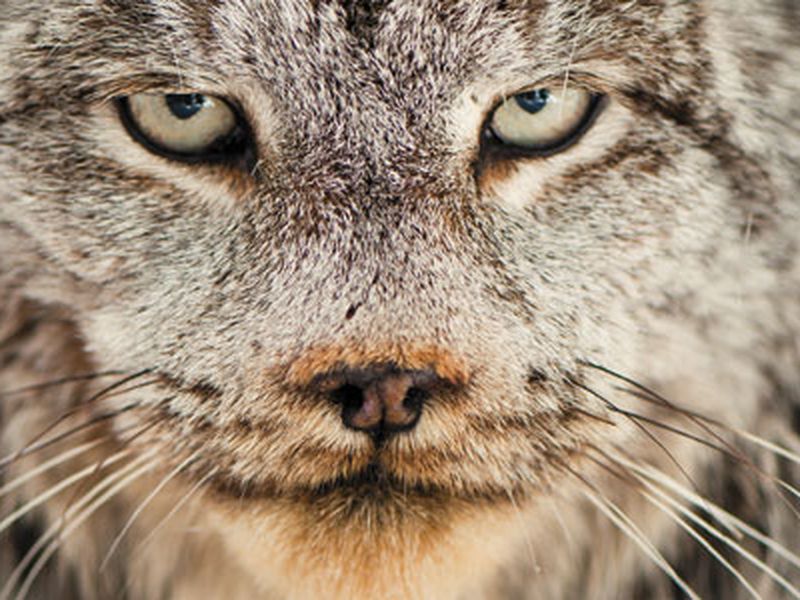This color photograph features an intense close-up of a mountain lion or puma, capturing its face from just below the chin to just above the eyes. The entire frame is filled with the cat's head, highlighting its steely, pale yellow eyes that seem to scrutinize the viewer with a no-nonsense expression. The mountain lion's fur displays a mix of brown, black, tan, and white shades, with notable orange smudges above its nose that resemble spray paint. Prominent black and white whiskers extend from each side of its snout. The creature’s gaze is intense, and its slightly squinting eyes convey a wild and somewhat mean look, underscoring its untamed nature. The close-up view, emphasizing the animal's facial features, offers a striking and detailed portrait of this majestic big cat.